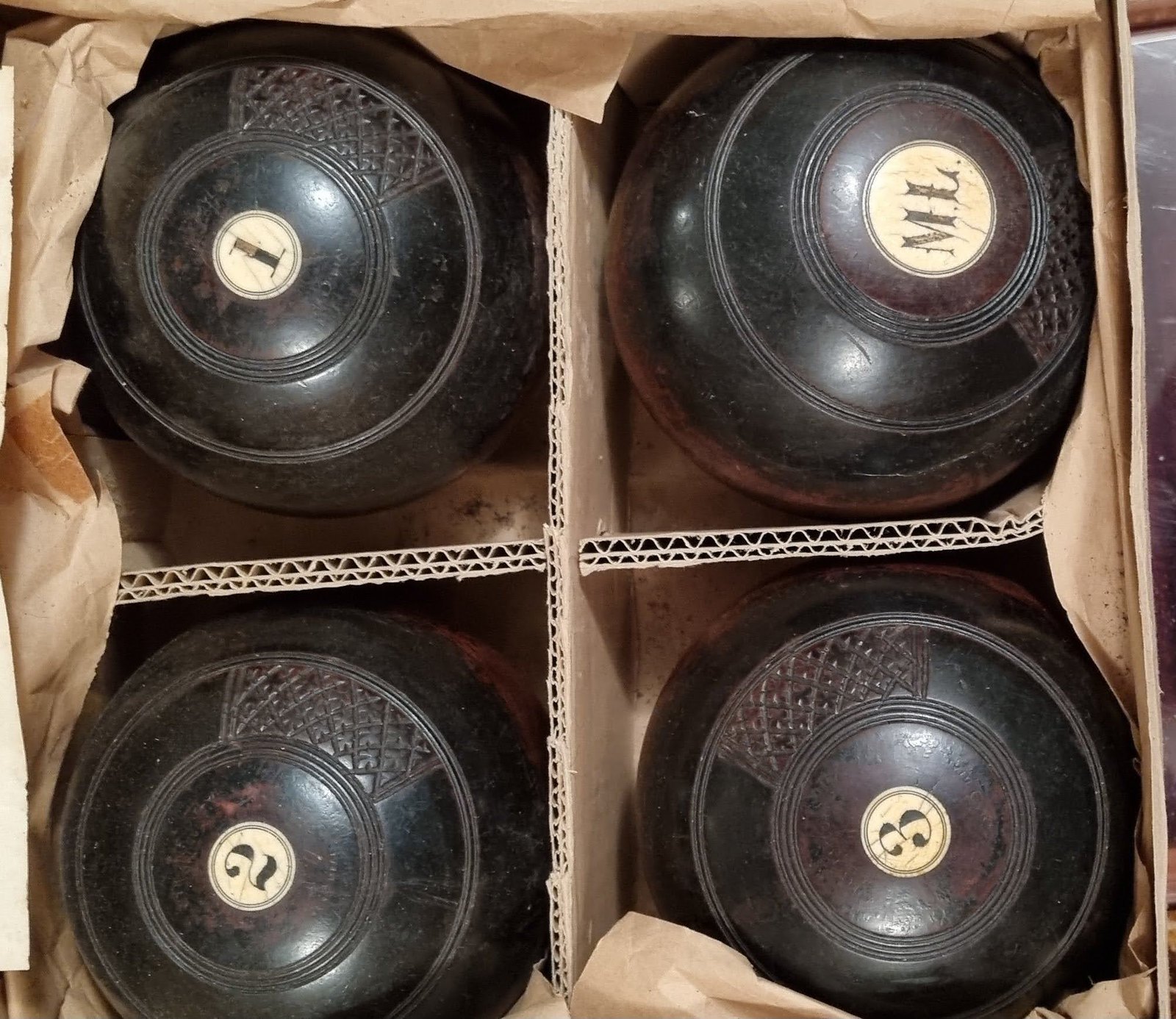This color photograph offers a detailed top-down view of a cardboard box divided into four compartments by corrugated cardboard partitions. Each compartment contains a black, spherical object that appears somewhat aged and scratched. These spheres are marked by concentric circles at their centers, each featuring distinct labels: '1' in the top left, 'ML' in the top right, '2' in the bottom left, and '3' in the bottom right. The objects are cushioned with protective tissue paper and have some chocolate brown accents. Although they resemble balls such as cue balls or eight balls, their exact nature is ambiguous. Their polished, almost stone-like appearance contributes to the mystery of their purpose.